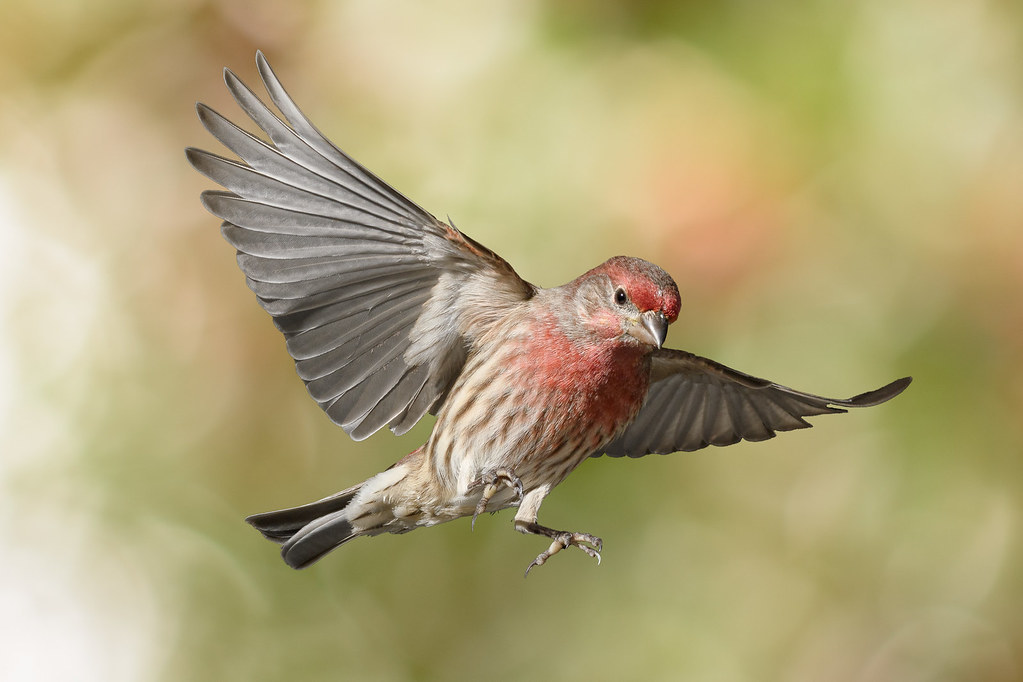This is a stunning close-up photograph of a bird in mid-flight, showcasing its intricate details and vibrant colors. Its outstretched wings are a striking blend of gray and gray-brown, each feather beautifully defined. The bird's head is predominantly gray with a notable red forehead that seems to encircle its head. Its sharp gray beak and the single visible black eye give it a determined look. The throat displays a striking red that extends down to its chest, which is adorned with vertical brown and white stripes. Its legs are extended, preparing for a landing, with claws splayed open. The bird's tail is also outstretched, showing light brown and white hues with horizontal brown stripes leading to the feathers. The background is artistically blurred with hues of green, red, and pink, adding to the overall mystique and beauty of the image.